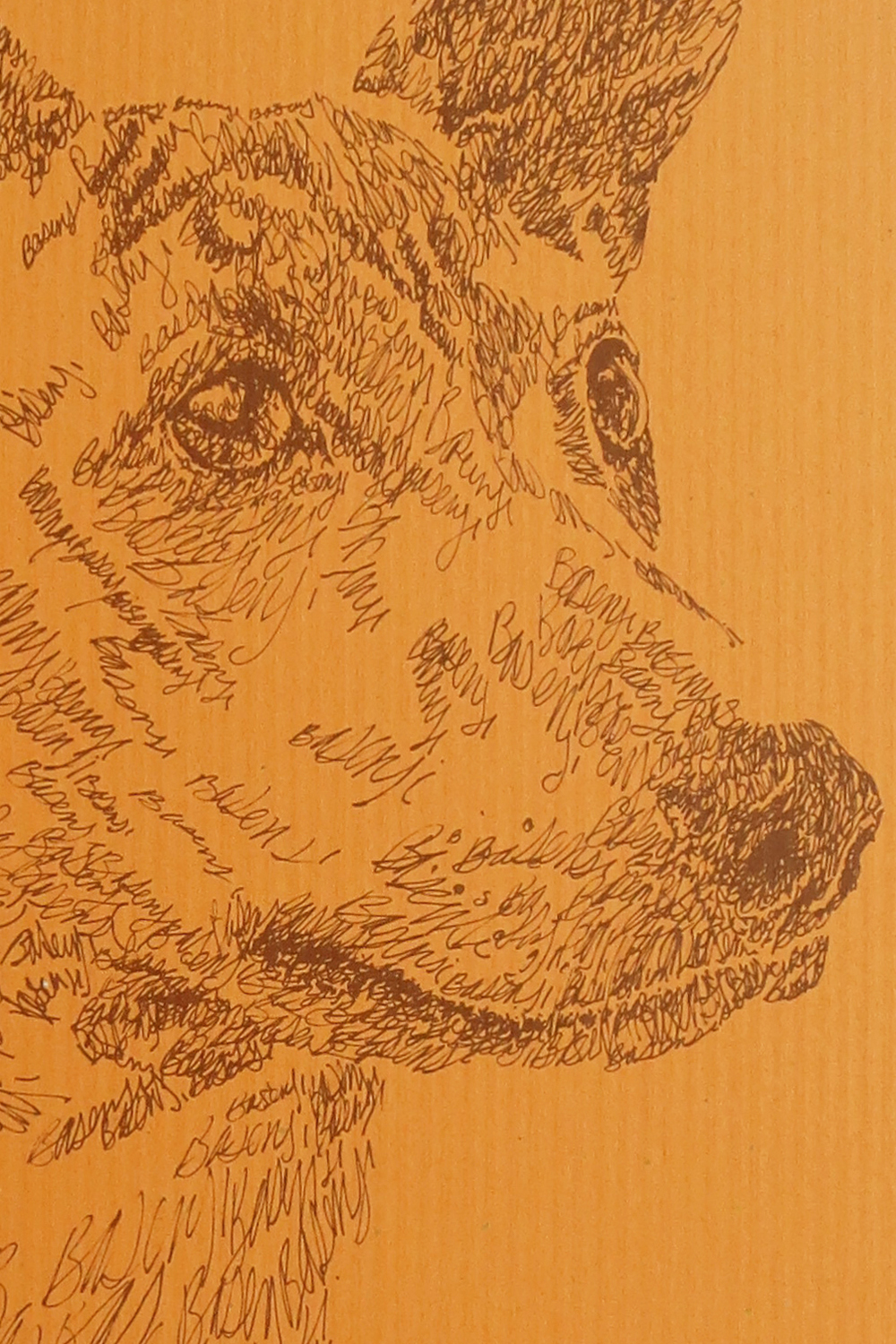This artwork is an artistic rendering of a dog's profile, primarily focusing on the facial features such as the eyes, nose, and ears. The style is notably unorthodox and scribbly, composed of dark, possibly brown pen-like lines, meticulously placed to convey the dog's appearance without a traditional outline. The dog seems to have pointy ears and a larger snout, with details particularly emphasized around the eyes and nose areas. The background is an orange or light brown tinted paper, reminiscent of cardboard or construction paper, adding to the rustic aesthetic of the piece. Despite the sketchy and scribbly style, the artwork is richly detailed. There's a special touch with what appears to be the name of the dog subtly included in cursive within the details, hinting at characters like 'B' and 'Y'. The portrait mostly features the dog's face in profile, with a hint of its chest area visible.